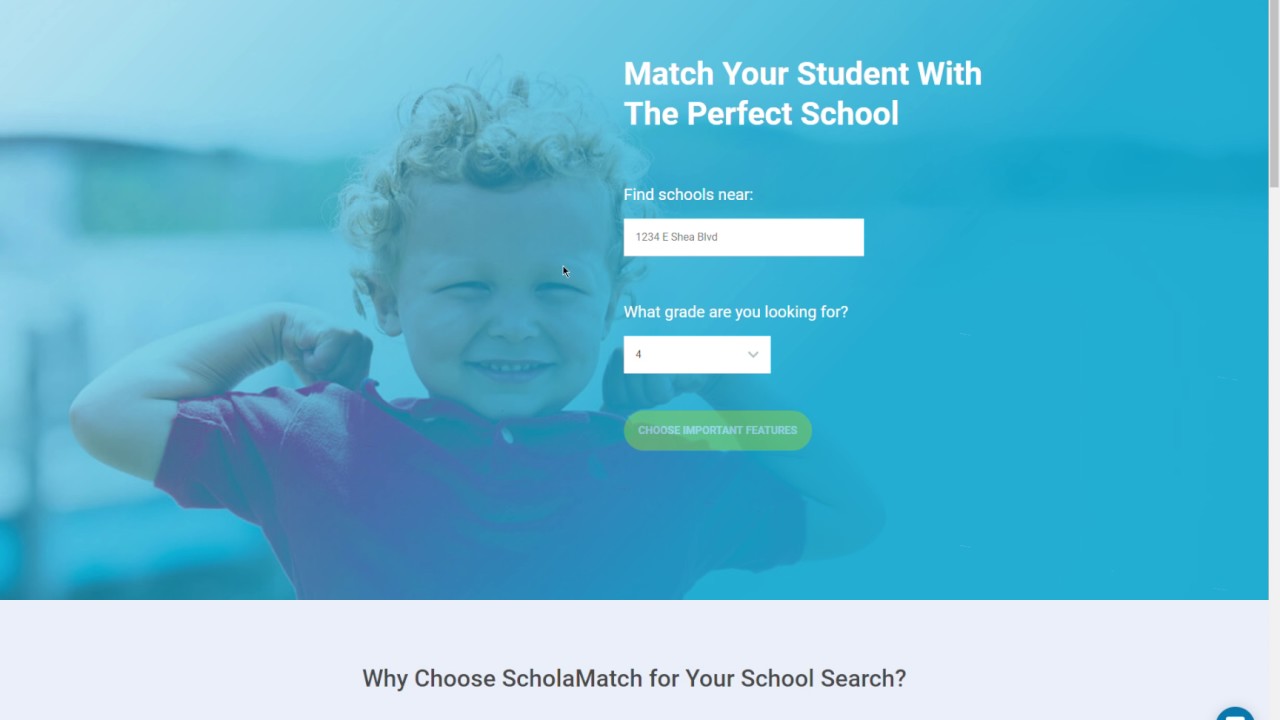The webpage, designed to help parents match their children to suitable schools, features a vibrant teal background. Dominating the background is a cheerful image of a young boy, approximately five or six years old. He is smiling widely, flexing his arms in a playful bodybuilder pose. The boy, who has short, curly blondish-brown hair and fair skin, is dressed in a dark reddish-purplish t-shirt.

At the top of the page, bold text reads, "Match Your Student with the Perfect School." Beneath this heading, a prominent white input box invites users to "Find Schools Near You." Within this box, there's a placeholder for entering an address, indicating that users can search for schools based on their specific location.

Below the address input, a dropdown menu prompts the user to select a grade level, currently set to fourth grade. This tool allows further refinement of the search based on the student's grade level. 

Further down, a greenish button with white text reads, "Choose Important Features." This button likely opens additional filtering options, enabling users to tailor their search with specific attributes and criteria important to them.

The page also includes a section titled, "Why Choose School of Match for Your School Search?" which presumably provides explanatory information and benefits about using this matching service.